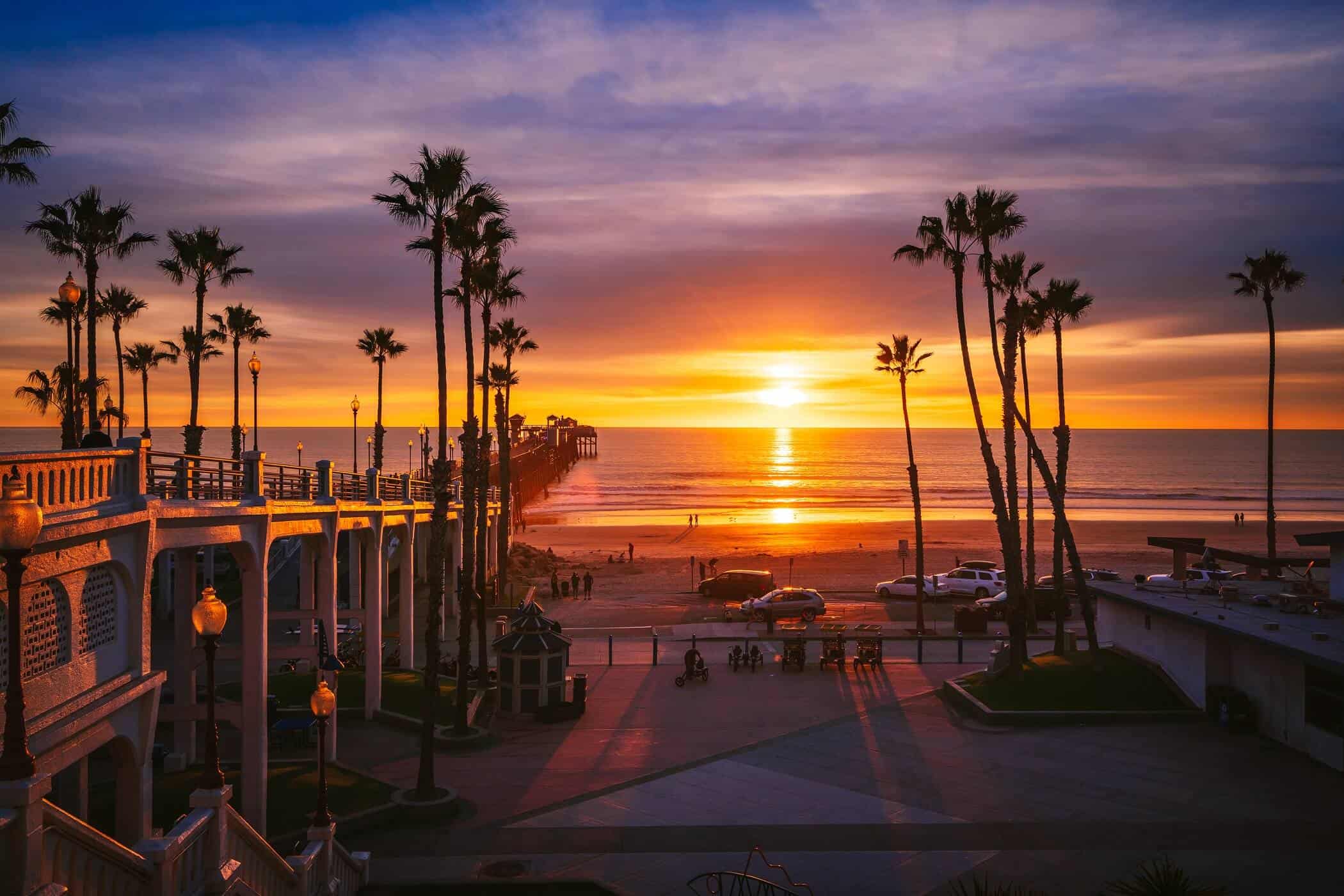This captivating sunset photograph taken from a coastal vantage point features a picturesque beachfront scene. In the foreground, a stone courtyard area is prominent, bordered by a road that separates it from the sandy beach beyond. On the left side of the image, a pier extends over the courtyard and reaches out over the water, creating an engaging visual pathway into the ocean. Adjacent to the pier, numerous tall palm trees stand majestically, lining the left side of the view.

The sky is a breathtaking gradient, transitioning from a bright, glowing sun at the horizon through a spectrum of orange, purple, and finally to deep blue at the top. The sun's illumination casts a rich palette on the ocean, which mirrors the vibrant hues of the sky. Farther out, people appear as tiny silhouettes against the glowing backdrop, adding scale and life to the serene scene.

To the right, a small building is nestled among more palm trees, further adding to the tropical ambiance. Additional details include a row of horizontally parked cars near the beach and car stopper bars alongside the road, hinting at a well-visited spot. The stairs with railings near the beach suggest easy access for people making their way down to the shoreline. Overall, the image is an exquisite blend of natural beauty and subtle human activity, captured in the magical light of dusk.